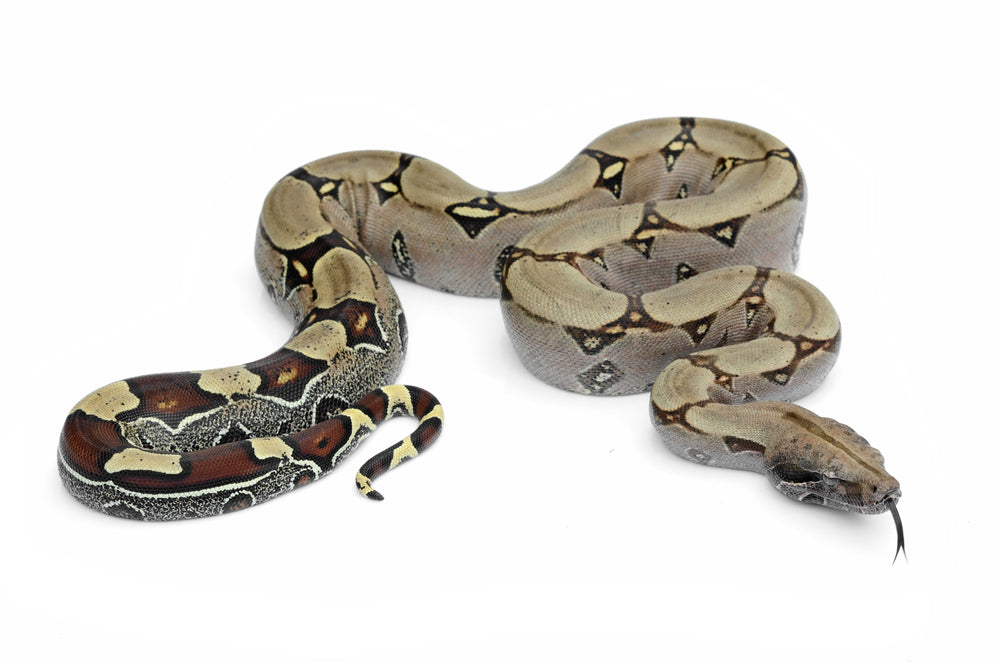The image features a close-up of a snake against a completely white background, which could either be a white surface or digitally altered to appear so. The snake is curled up, showcasing its intricate pattern and texture. Its body displays a gradient of colors, starting with a light greenish-gray hue near the head that transitions into darker shades as it moves toward the tail. Striking triangular and splotched patterns cover its body, with the coloration shifting from gray and black near the head to darker brown and reddish-brown tones toward the tail. The snake's forked tongue is captured mid-flicker, adding a dynamic element to the picture. The eyes appear almost white, with a distinctive black line running through the center. Overall, the snake’s patterned appearance and varying colors suggest it could easily blend into a rocky environment.